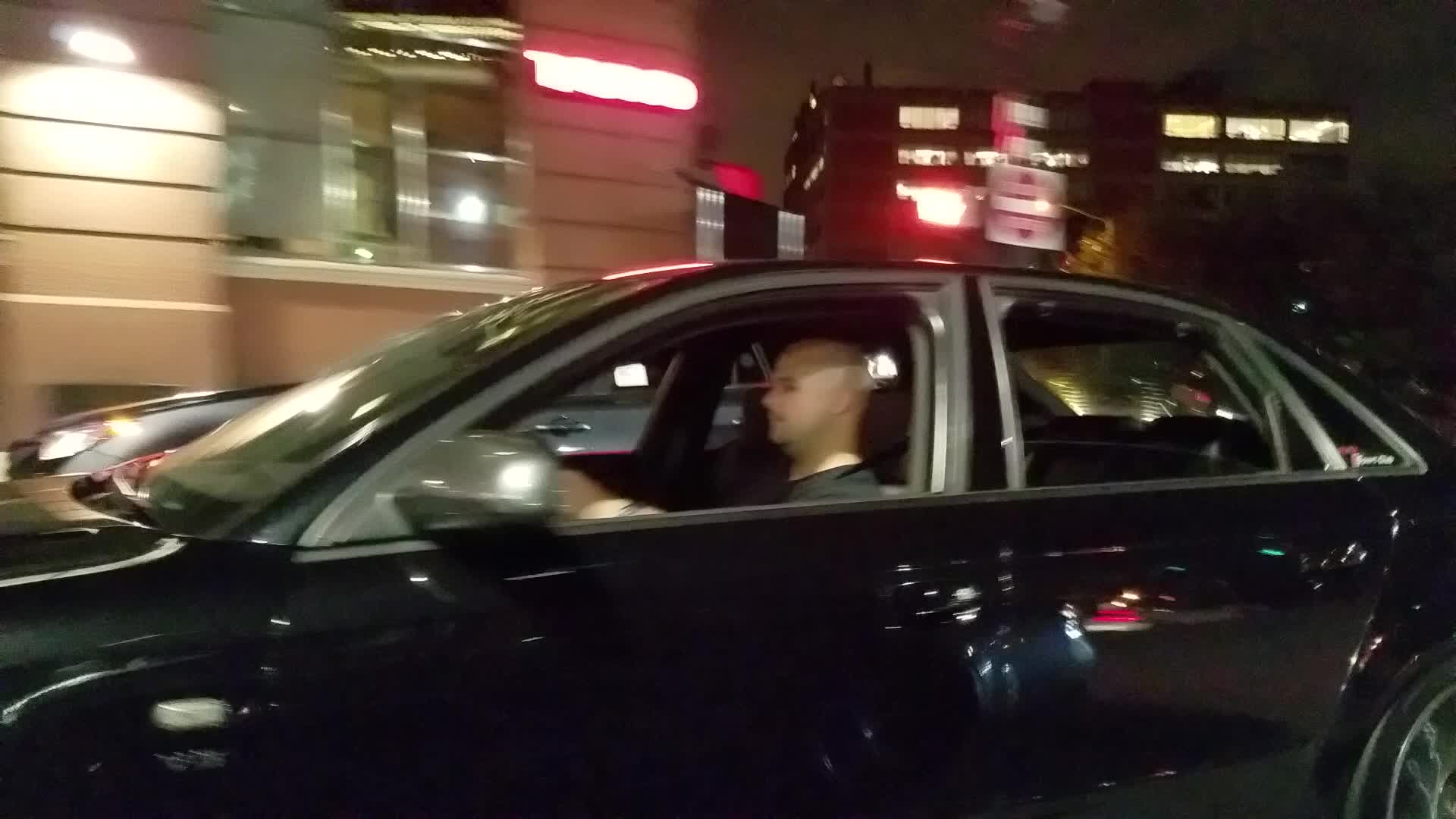A photo taken from the passenger side of a vehicle captures a bustling nighttime scene on a multi-lane road. The focus of the photograph is a black, four-door car in the adjacent lane, very close to the photographer's vehicle, which reflects in the black car's door. The driver of the black car, a bald man in a black t-shirt, is seen through his open windows, staring straight ahead. Through these windows, a silver car in the background is also visible. In the top-left corner of the image, a building with a small red neon sign is positioned close to the road, while the top-right corner reveals the silhouettes of taller buildings farther away. A blurred road sign indicates the movement of vehicles, accentuating the busy urban landscape. The dark night sky frames the scene, highlighting the contrast with the illuminated elements.